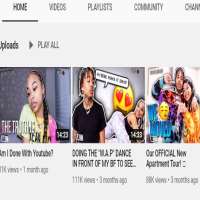The image appears to be a pixelated and zoomed-in screenshot of a YouTube channel page. The main section visible is labeled "Uploads Play All," suggesting it displays recent video uploads. There are three video thumbnails discernible in the screenshot. The titles of the videos are as follows: "Am I Done with YouTube?" dated from a month ago, "Doing the WAP Dance in Front of My Boyfriend to See His Reaction," and "Our Official New Apartment Tour," both uploaded three months ago.

The YouTube channel seems to belong to a vlogger who shares various aspects of their personal life, including pranks and day-to-day experiences with their boyfriend. The title of the most recent video, "Am I Done with YouTube?" hints at a potential hiatus or break from creating content, which is a common practice among vloggers who often return to explain their absence to their subscribers.